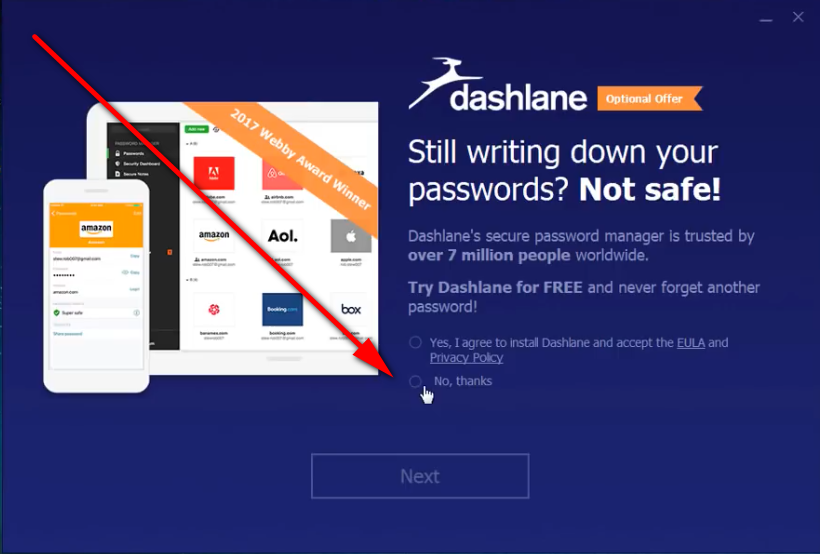The screenshot captures a website with a dark blue background that transitions from a deep navy at the top to a lighter, brighter blue towards the bottom. 

In the top right corner, there is a small line next to an 'X,' likely representing a close button. On the top left, a filled-in red arrow diagonally points towards the center of the screen. Below this arrow, to the left, is a banner with a white background framed by an orange border that reads "2017 Webby Award Winner."

Beneath this banner, there is a white drawing of a cell phone with an orange background. The text "Amazon" appears on the cell phone, although additional details are difficult to read. This area highlights various websites, including AOL, Box, and Amazon.

Outside this white banner area, on the blue background, a deer is shown leaping with the text "DASHLINE" nearby. Below the leaping deer, an orange banner states: "Optional Offer" followed by the message "Still writing down your password? Not safe!" in a lighter font and "DASHLINE Secure Password Manager is trusted by over 7 million people worldwide" in a bolder font. It encourages users to "Try DASHLINE for free and never forget another password," with "free" emphasized in uppercase letters.

Further down, there are buttons for user interaction: "Yes, I agree to install DASHLINE, accept the privacy policy," and "No thanks," the latter accompanied by a pointing hand icon. Finally, the word "Next" appears in light gray text within an outline.